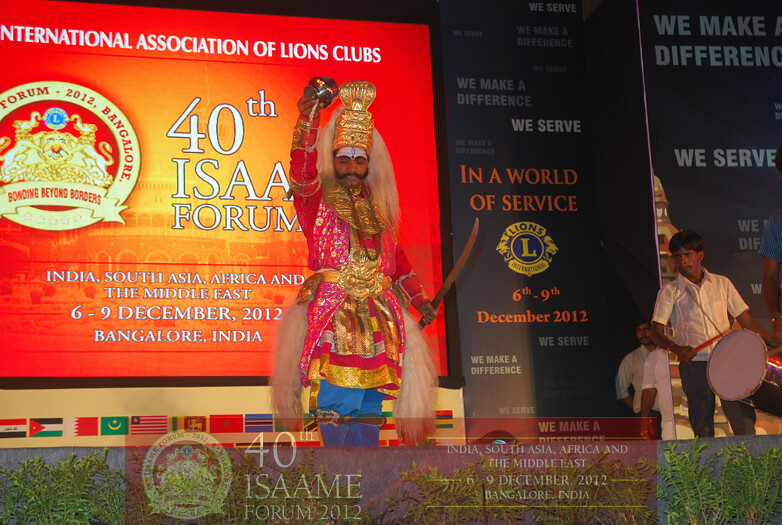The image captures a richly adorned man standing at the center front of a stage, dressed in an elaborate ceremonial costume. He wears a golden crown with white hair flowing out and a striking pink and gold outfit resembling a dress with a large gold belt. His ensemble features intricate flower patterns, gold bands, and a royal blue undertunic. A distinctive long mustache graces his face, and he wields a curved sword in one hand while raising a golden-gloved fist in the air. Additionally, he has long hair on either side of his legs. Behind him, a projector screen displays the text: "International Association of Lions Clubs 40th ISAA India, South Asia, Africa, and the Middle East, 6 to 9 December 2012 Bangalore, India." A man playing a drum is positioned to the right in the background. The vibrant scene is composed of colors such as red, blue, green, white, black, and gold.